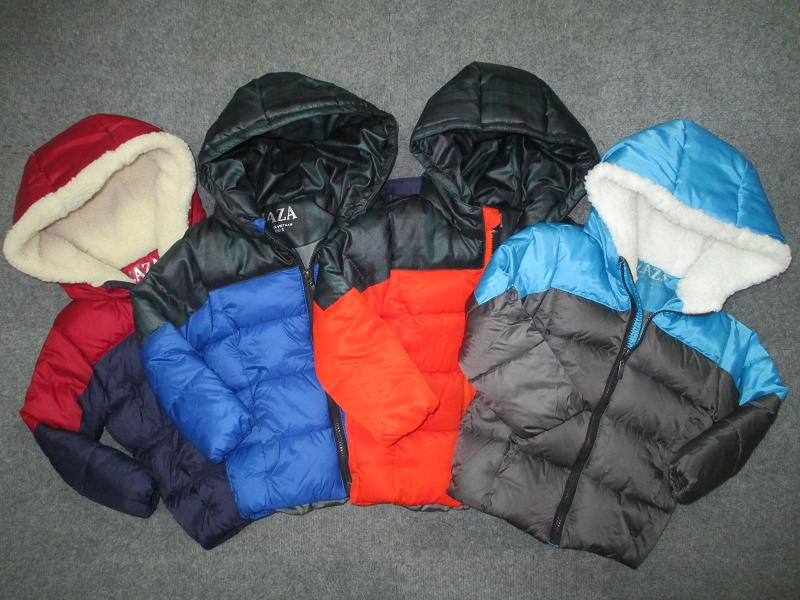In this top-down image, four child-sized puffer jackets are arranged in a horizontal curve on a gray carpeted floor. All the jackets have hoods and appear to be for small children, roughly ages two to five. They overlap each other halfway, showcasing their vibrant colors and designs. From left to right, the first jacket is a red and dark blue combination with a furry cream-colored lining; the second is blue and black with a black hood and silky lining. The third jacket features a black hood with an orange bottom and a black lining, while the last one is a light blue and dark gray jacket with a hood lined in soft white fur. Each jacket is poofy with horizontal ripples, and their labels, where visible, read "AZA."